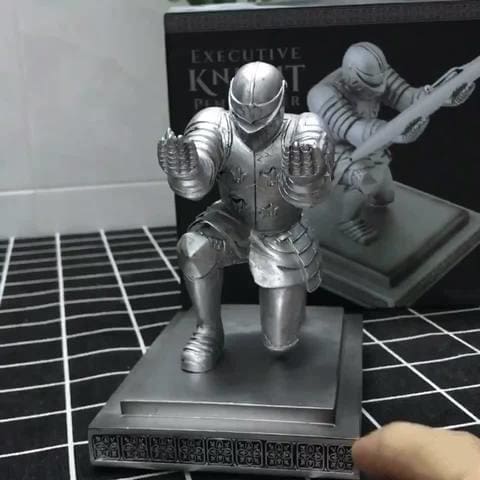This image showcases ornate silver knight statuettes. Each knight is dressed in detailed armor, exuding a sense of historical regality. The statuettes rest on rectangular bases colored in a dark gray hue, adorned with intricate, potentially floral, patterns along the sides. These ornate designs highlight the craftsmanship and attention to detail. The base features an additional raised rectangular section, slightly smaller in dimension, enhancing the elegance of the presentation.

The packaging of the statuette also displays an image of a knight and bears the text "Executive Knight." One knight statuette is positioned outside of its packaging, prominently displayed on a black and white tiled surface, likely a floor or counter. The composition of the image accentuates both the artistic and historical significance of the knight statuettes, making them stand out vividly against the monochrome background.